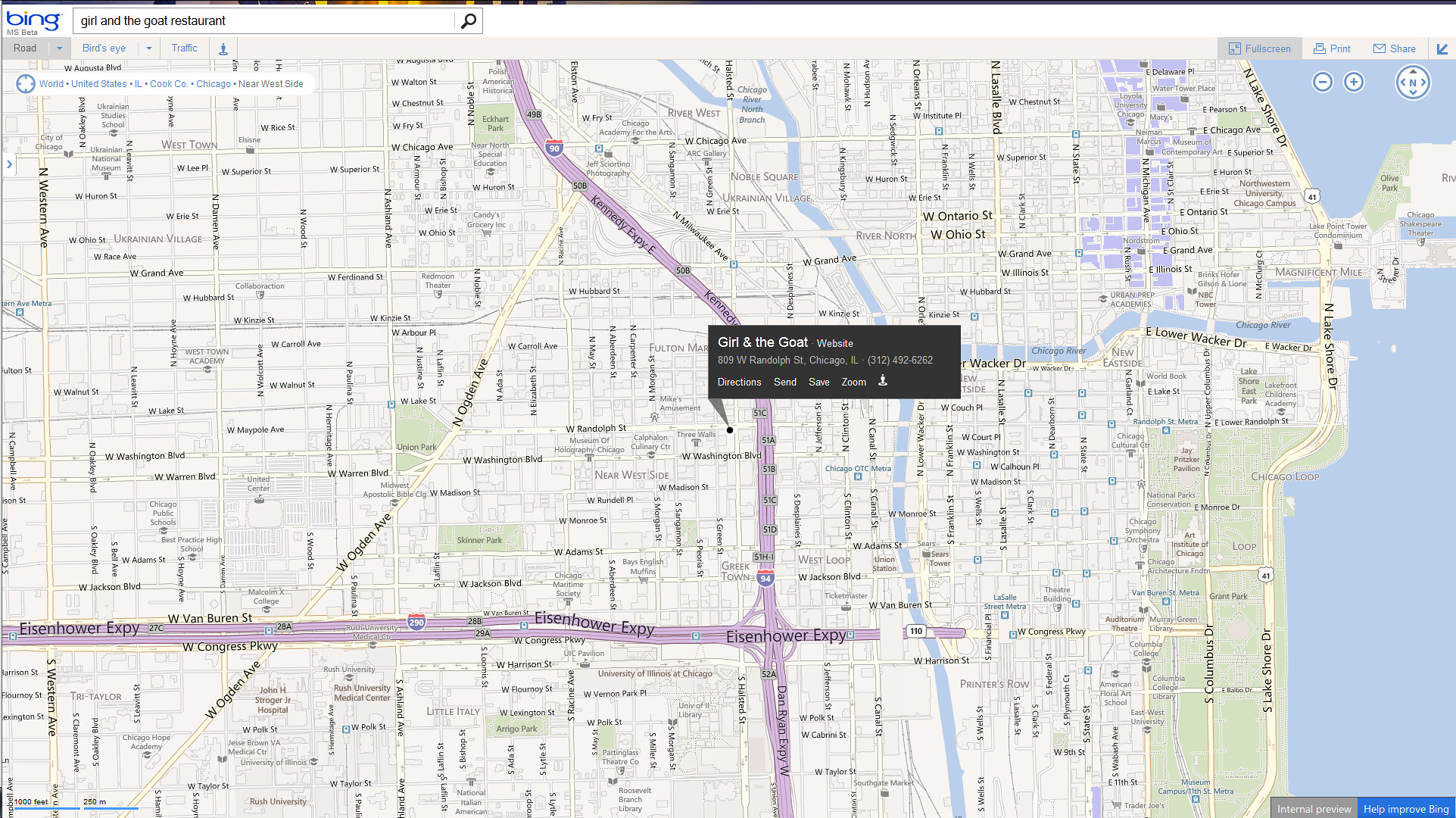This image is a screenshot of a Bing Maps search result for a location. At the top of the interface, a prominent white search bar is displayed, bearing the typed query "Girl and the Goat Restaurant." The Bing logo, colored in blue, is located in the top left corner of the screen. Adjacent to the search bar on the right, there is another empty input bar.

In the center of the map, a black popup bar highlights the location of the "Girl and the Goat" restaurant. This bar not only names the restaurant but also includes additional information and options such as saving the location or downloading details. The map itself showcases various streets and place names surrounding the restaurant, with the right side of the map featuring a body of water. Navigation controls, allowing the user to zoom in and out, are situated in the top right corner of the screen. The entire setup provides a comprehensive view of the restaurant's location and the surrounding area, ensuring users can easily find and explore "Girl and the Goat."